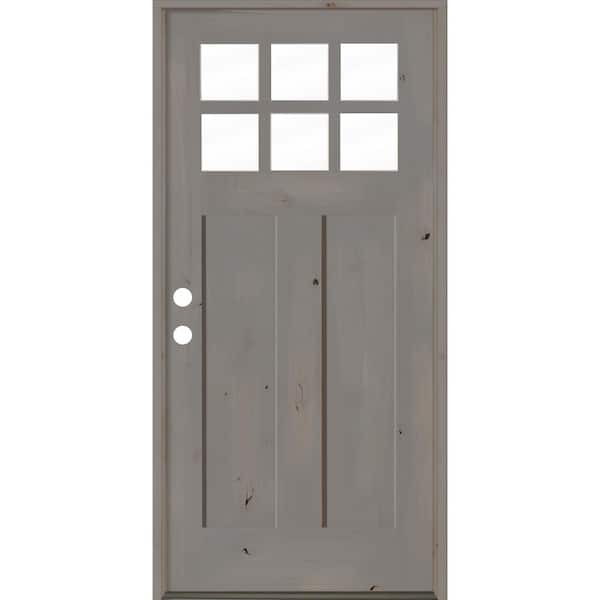This image features an unfinished gray-washed wooden door with a slightly distressed appearance. The door stands approximately 72 inches high and has a modern design with two main sections. At the top, there is a window divided into six square panes, without any glass, showing only a white background. Below the window, the door is adorned with two vertical panels that add to its aesthetic appeal. The door lacks a doorknob, evident from the two holes where the doorknob and deadbolt should be. Surrounding the door is a door jamb, and the wood showcases natural knots, emphasizing its wooden construction.